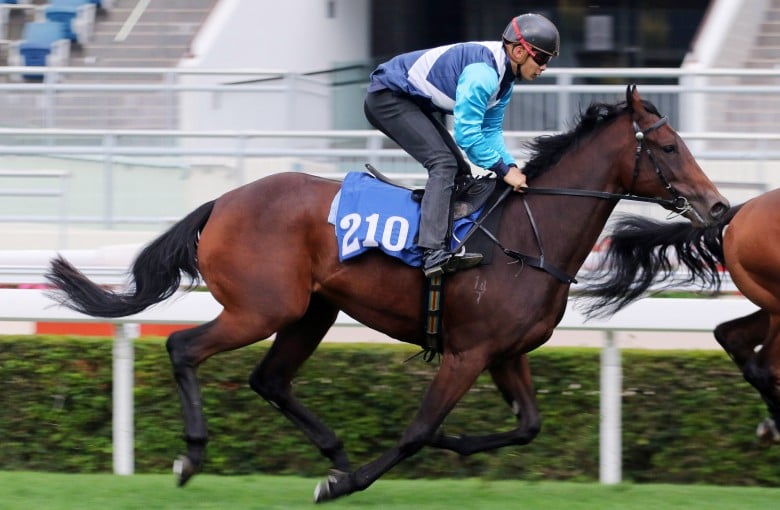This photograph captures a thrilling moment of a horse race in broad daylight, featuring a dark chestnut racehorse with a black mane and tail. The horse's legs transition from dark brown at the top to almost pitch black from the knees down, highlighting its sleek and powerful build. The racehorse, identified with the number 210 on a blue cloth under the saddle, is captured in full stride, indicating its rapid speed with legs positioned dynamically. 

Riding the horse is a jockey, slightly elevated off his seat, demonstrating his control and skill. He is outfitted in dark blue pants and a long-sleeve shirt in different shades of blue, with distinctive white chevron patterns adorning the sides. His black helmet with a pair of goggles strapped with red sits firmly on his head, projecting focus and determination. 

The scene is set on a grass track, bordered by a low hedge and a rail, with a glimpse of the spectator stands in the background, blurred slightly due to the speed at which the horse is moving. A few spectators are visible on the left side of the image, enjoying the race under a mildly sunlit sky, adding to the lively ambiance of this horse racing event.